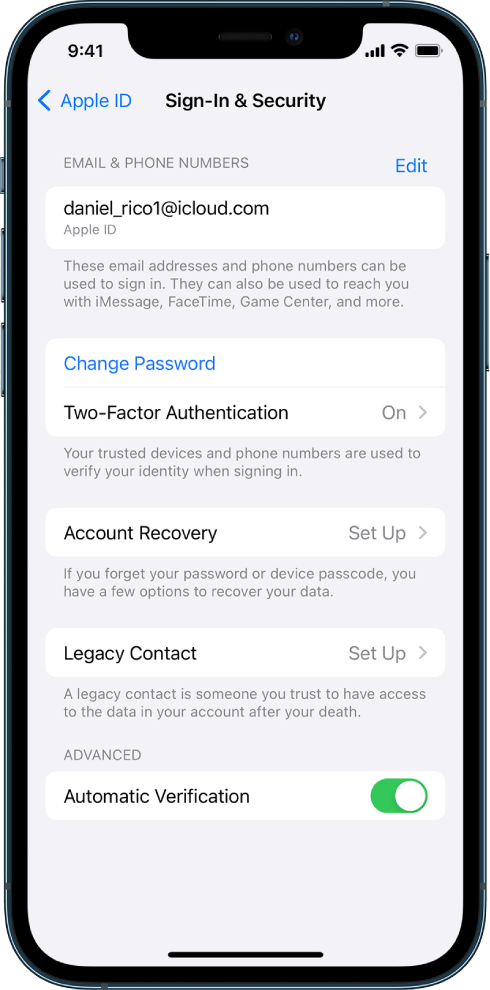The image depicts a smartphone with a sleek design characterized by a silver-colored outer edge and a contrasting black interior border. At the top of the black border, there is a small microphone or speaker opening alongside a circular camera lens. The left-hand side of the phone features three protruding buttons, while the right-hand side has a single large button.

The screen displays a gray-background interface showing the time as 9:41. There are icons indicating the status of data, Wi-Fi, and battery life. The screen is focused on the "Apple ID" settings section, specifically on "Sign-In and Security" and "Email & Phone Numbers." This section includes an editable entry for the Apple ID, listed as daniel__rico1 at iCloud.com, which can be used for signing in, as well as for iMessage, FaceTime, Game Center, and other services.

Below, there is an option to change the password, highlighted in blue, along with a notification that two-factor authentication is enabled. Additionally, there is a setup option for account recovery, offering various methods to retrieve account credentials if the password or passcode is forgotten. The settings also mention "Legacy Contact," allowing a trusted individual access to account data after the owner's death. The "Advanced Automatic Verification" option is toggled on, indicated by a green switch.